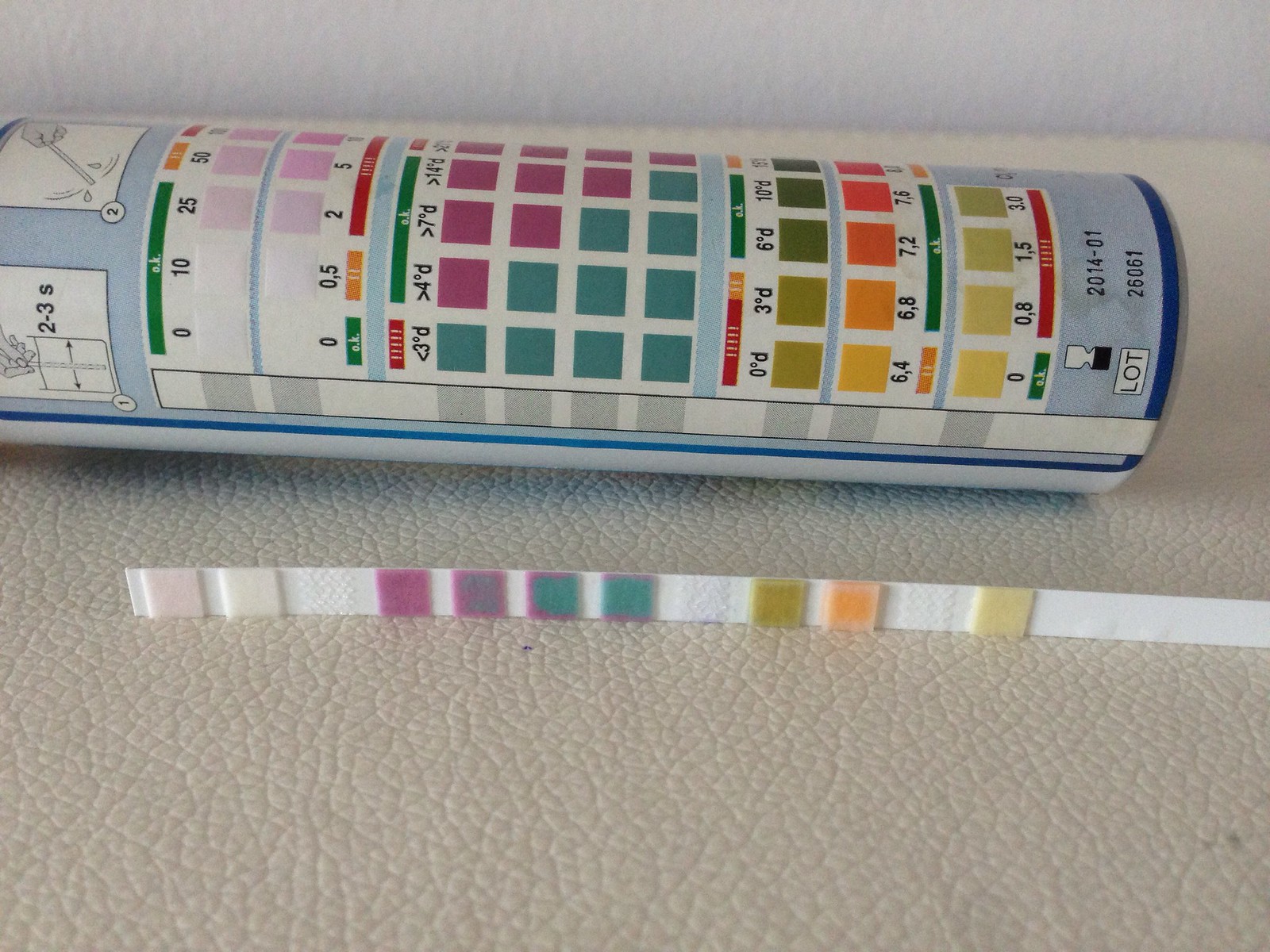The image showcases an oblong canister placed on a table with a white, bumpy texture. The canister appears to be designed for pH testing, displaying a detailed pH color chart. Each strip on the canister features a series of colored squares, progressing from white on the left, through shades of purple and blue, and finally to greenish-yellow, peach, and beige on the right. These colors correspond to varying pH levels, indicating the level of acidity or basicity of a substance. A strip, identical to the ones shown on the canister, lies next to it, offering a real-world example. The colors on the strip include two white squares, followed by gradual changes from purple to blue, and ending with light greenish-yellow, peach, and beige squares. Each color on the canister is paired with specific pH numbers below it, helping to interpret the pH level accurately. The base of the canister is marked with a date, "2014-01" or possibly "2014-07," depending on the viewing angle, along with a lot number for tracking.